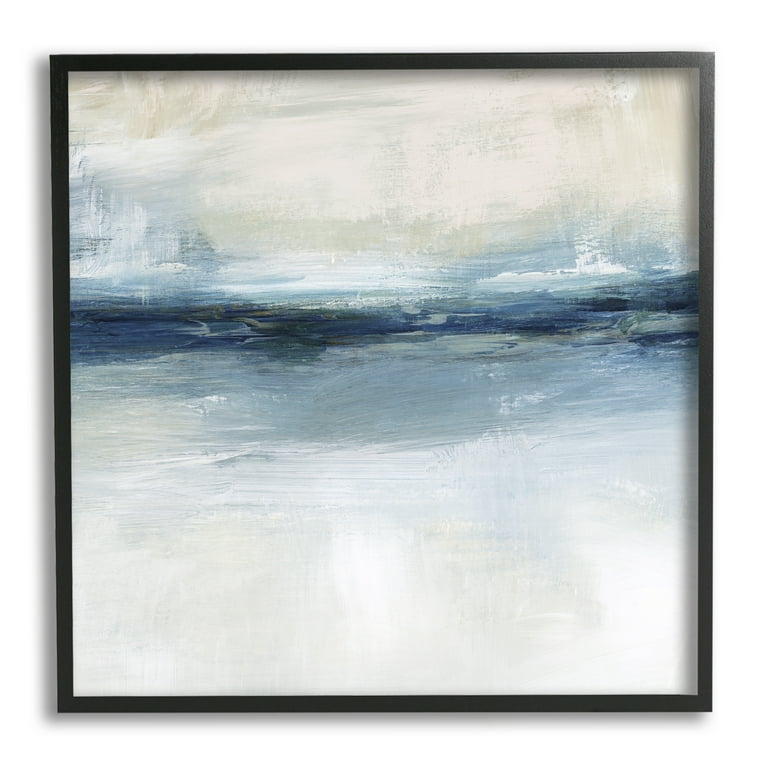This is an image of an abstract painting set within a thin black matte frame, likely made of wood or plastic. The painting predominantly features an ocean theme, depicted through a progression of colors across the canvas. At the bottom, the painting is mainly white, possibly representing reflections on water or snow. This white area transitions gradually into a light blue, then into a darker bluish-gray section, which occupies the majority of the canvas and suggests deeper water. Near the middle, a prominent dark blue horizontal line stretches from one edge to the other, indicating the horizon or a deeper part of the ocean, with a mixture of lighter blues interspersed, simulating waves or splashes of water. Toward the top, the colors shift to off-white and beige hues, which may symbolize the sky or distant landmasses. The painting's brush strokes vary, with the blue tones executed in horizontal motions, contrasting with the vertical strokes of the whites. A subtle reflection on the top-right corner of the frame hints at an external light source. The overall composition, while simple, evokes a serene oceanic or winter landscape, open to interpretation due to its abstract nature.